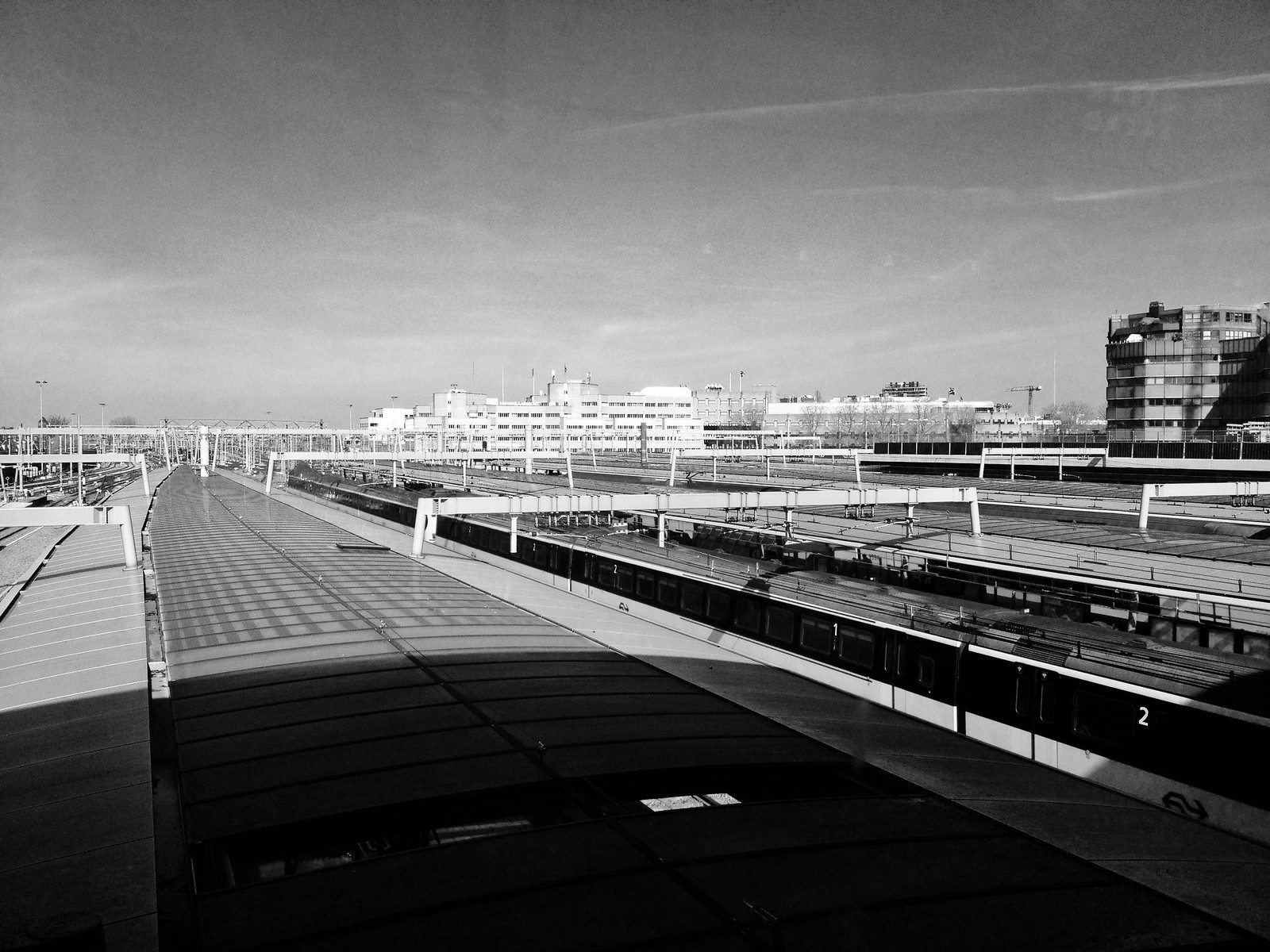The image is a black and white photograph capturing a detailed scene of a cityscape dominated by a sprawling train station in the foreground. Multiple trains are lined up on parallel tracks, with the tops of the trains and the distinct black strips of their windows contrasting against the lighter tones of their sides. The station features extensive roofing and structural elements, including white bars or brackets, adding depth and complexity to the scene. In the background, a variety of buildings rise, notably several apartment buildings that are wide and not particularly tall, except for one that stands out at around six or seven stories high. The skyline is relatively low, with a lightly clouded sky that darkens toward the top of the image, casting shadows along the extensive metal roof structures that stretch from the bottom of the frame into the distance. The interplay of light and shadow enhances the architectural and structural details, painting a vivid picture of urban life in monochrome.